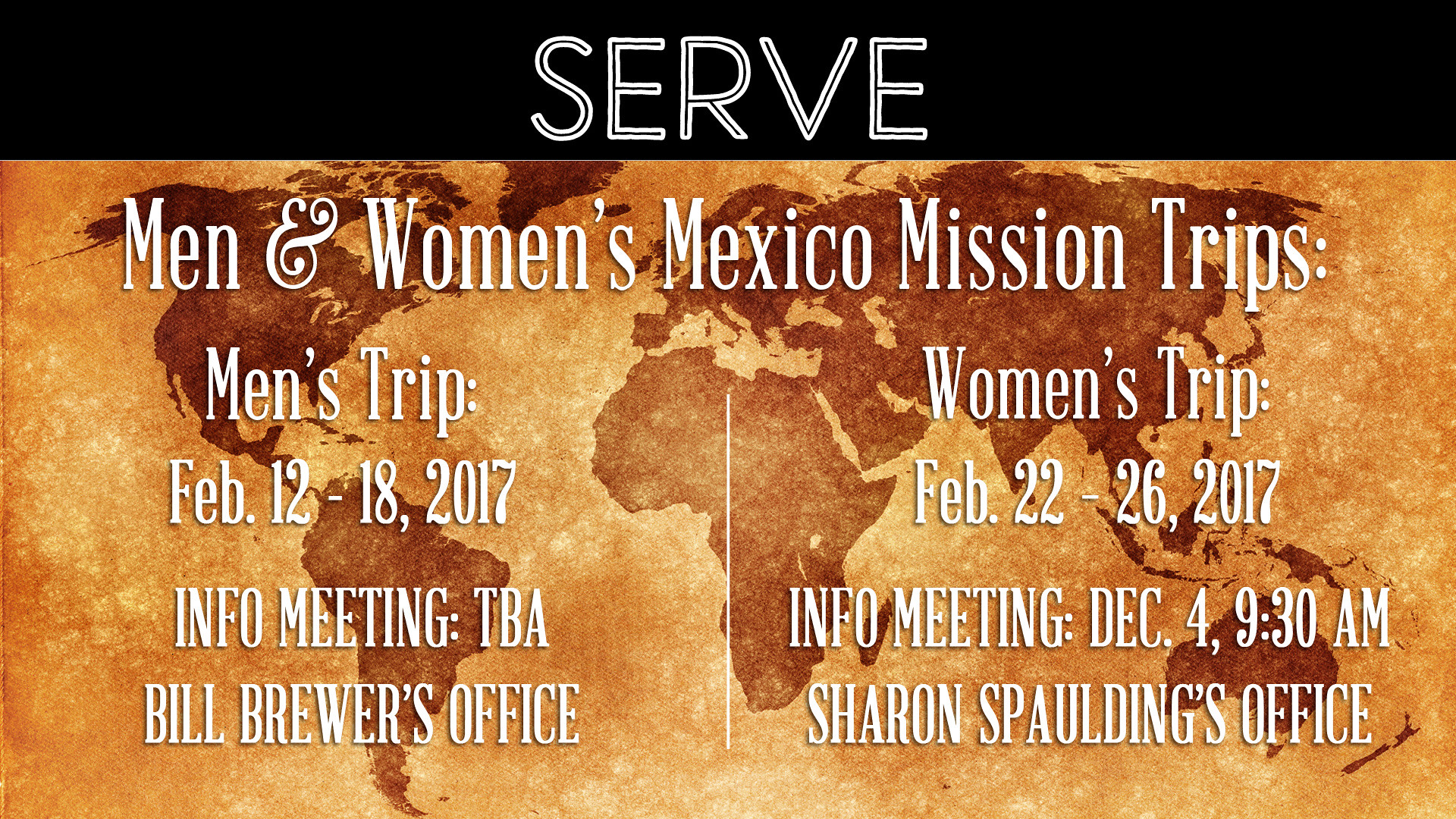The image features a rectangular banner with a prominent black border at the top, spanning from left to right, containing the white, all-capitals text "SERVE." Below this border is a sepia-toned world map showing various continents in shades of brown. Superimposed on the map in white text are the words "Men & Women's Mexico Mission Trips."

On the left half of the image, beneath the main title, detailed information about the men's trip is provided:
- Men's Trip: February 12-18, 2017
- Info Meeting: TBA at Bill Brewer's office

To the right of this, details for the women's trip are listed:
- Women's Trip: February 22-26, 2017
- Info Meeting: December 4, 9:30 AM at Sharon Spalding's office

The banner appears to be a print ad, likely for a Christian mission group, emphasizing the dates and details of these mission trips to Mexico. The text, primarily in white and thin, is highlighted against the dark and sepia background, making it clear and easy to read.